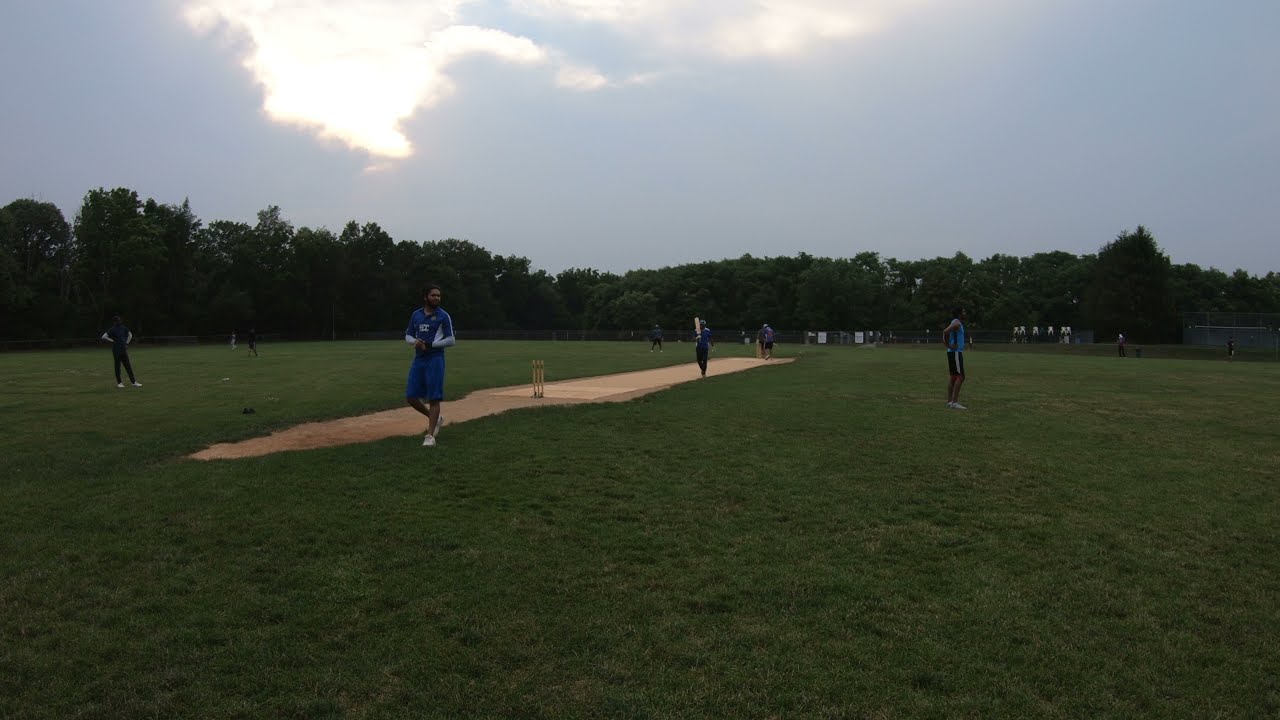The photograph captures a dynamic scene during a cloudy dusk on an outdoor cricket field. The field is expansive and predominantly covered in green grass, with a central rectangular pitch of sand and dirt, topped with three wooden stumps at one end. Various players in blue jerseys with white stripes and blue shorts are actively engaged in the cricket game, their white shoes striking against the green backdrop. Two batsmen stand on the pitch, each holding a bat and ready to play. Beyond the players, several spectators watch from near the boundary, lending a sense of community to the scene. Further in the distance, a metal chain-link fence adorned with multiple white posters separates the field from a dense tree line, where trees with dark green leaves create a rich, natural border. The sky is a mostly dark gray with heavy clouds, though a patch of light hints at the sun breaking through, adding a subtle contrast to this lively, outdoor scene.